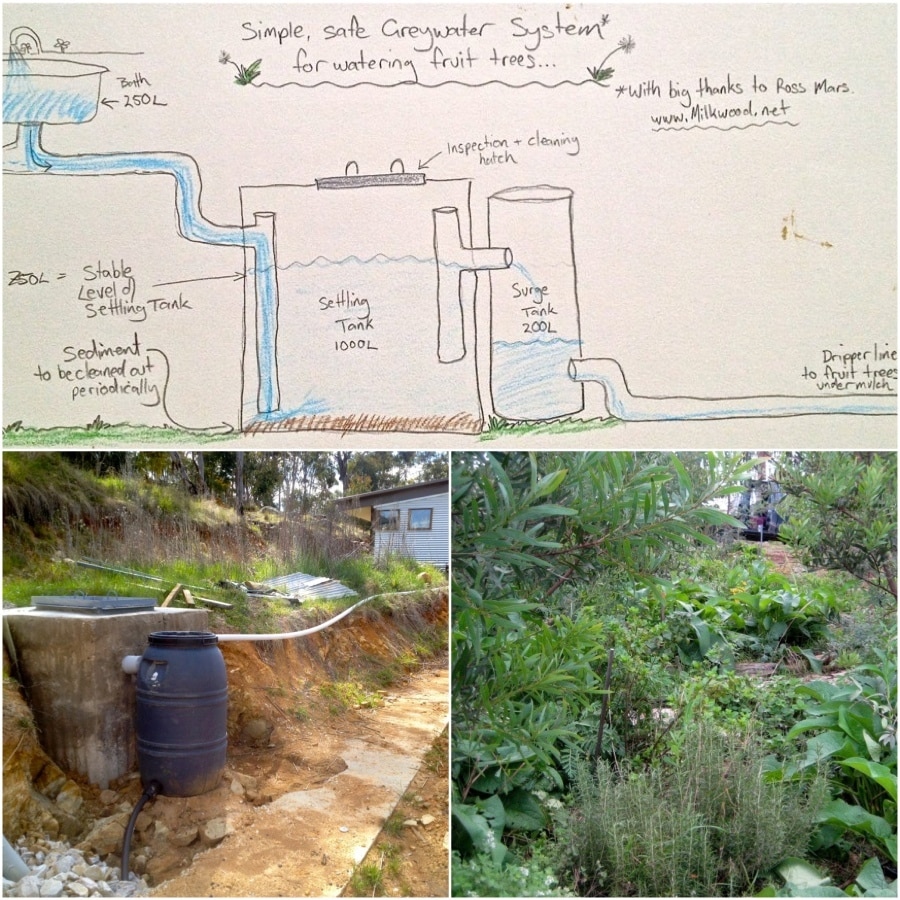The image is a detailed hand-drawn diagram titled "Simple Safer Greywater System for Watering Fruit Trees," with a big thanks to Ross Mars and the website www.milkwood.net mentioned below the title. The top half of the image illustrates the greywater system, which starts with bathwater (indicated as 250 liters) flowing through a series of pipes. The water first enters a settling tank with a stable level indication marked as 250 milliliters. This tank, which has a capacity of 1,000 liters, features an inspection and cleaning hatch on top. 

From the settling tank, the water moves through another pipe to a cylindrical surge tank, holding 200 liters. A pipe from this surge tank leads out to a dripper line that irrigates the fruit trees. 

Accompanying this detailed diagram are real-life photographs showing the components of the system: a concrete barrel acting as the settling tank, a smaller black barrel as the surge tank, and pipes extending towards the vegetation. In the background of the image, there are visible elements of a house, dirt, trees, and grass. The bottom left photograph depicts the system's layout, while the right photograph shows thriving plants irrigated by the greywater system.